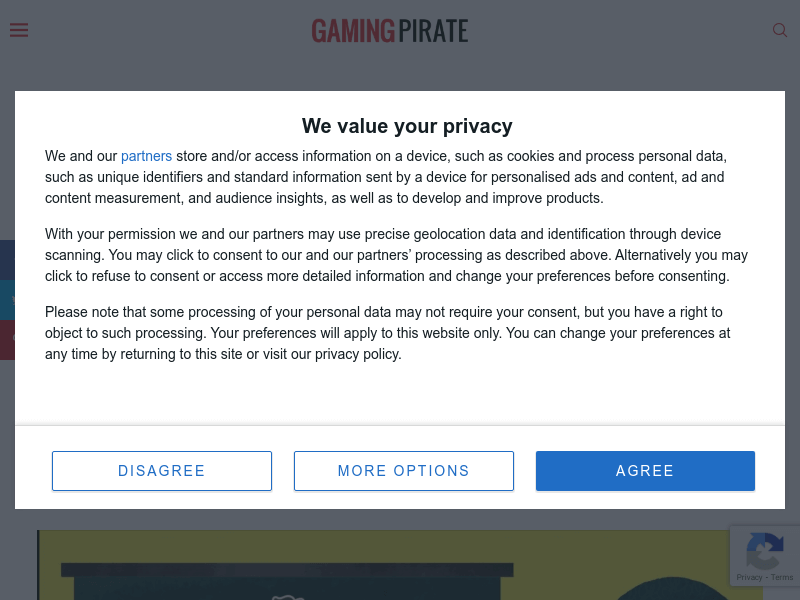The image captures a cookie consent pop-up on the GamingPirate website. The foreground prominently features a privacy notice that reads: "We value your privacy. We and our partners store and access information on your device, such as cookies, and process personal data. With your permission, we may use precise geolocation data to identify your device through scanning. You may click to consent. Please note that some processing of your data may not require your consent. You have the right to object.” Below this text, there are three buttons: "Agree," "Disagree," and "More Options," with no option to close the pop-up without making a selection. The background hints at the GamingPirate website content, though it is mostly obscured by the pop-up. The site’s name evokes curiosity, possibly suggesting either a playful take on a pirate-themed gaming site or a site that discusses the piracy of games.